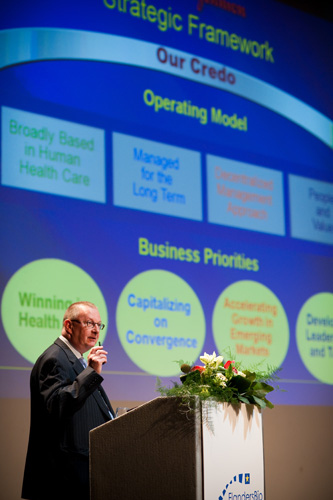An older white man with thin, graying hair and glasses stands at a light gray podium adorned with a bouquet of green leaves, white and red flowers. He's dressed in a black suit and white collared shirt. He holds a remote or pointer in his right hand as he presents to an audience. Behind him, a large, slightly blurry projector screen displays a PowerPoint slide with a blue background and yellow text at the top that reads "Strategic Framework: Our Credo, Operating Model." The screen features a series of rectangular text boxes outlining concepts such as "Broadly Based in Human Health Care" and "Managed for the Long Term," with additional blurry text. Beneath these, circular text boxes detail "Business Priorities," though the specific content is mostly indistinct. The podium also has a partially visible white poster with blue elements, and the image is captured from a side view, making some details less clear.